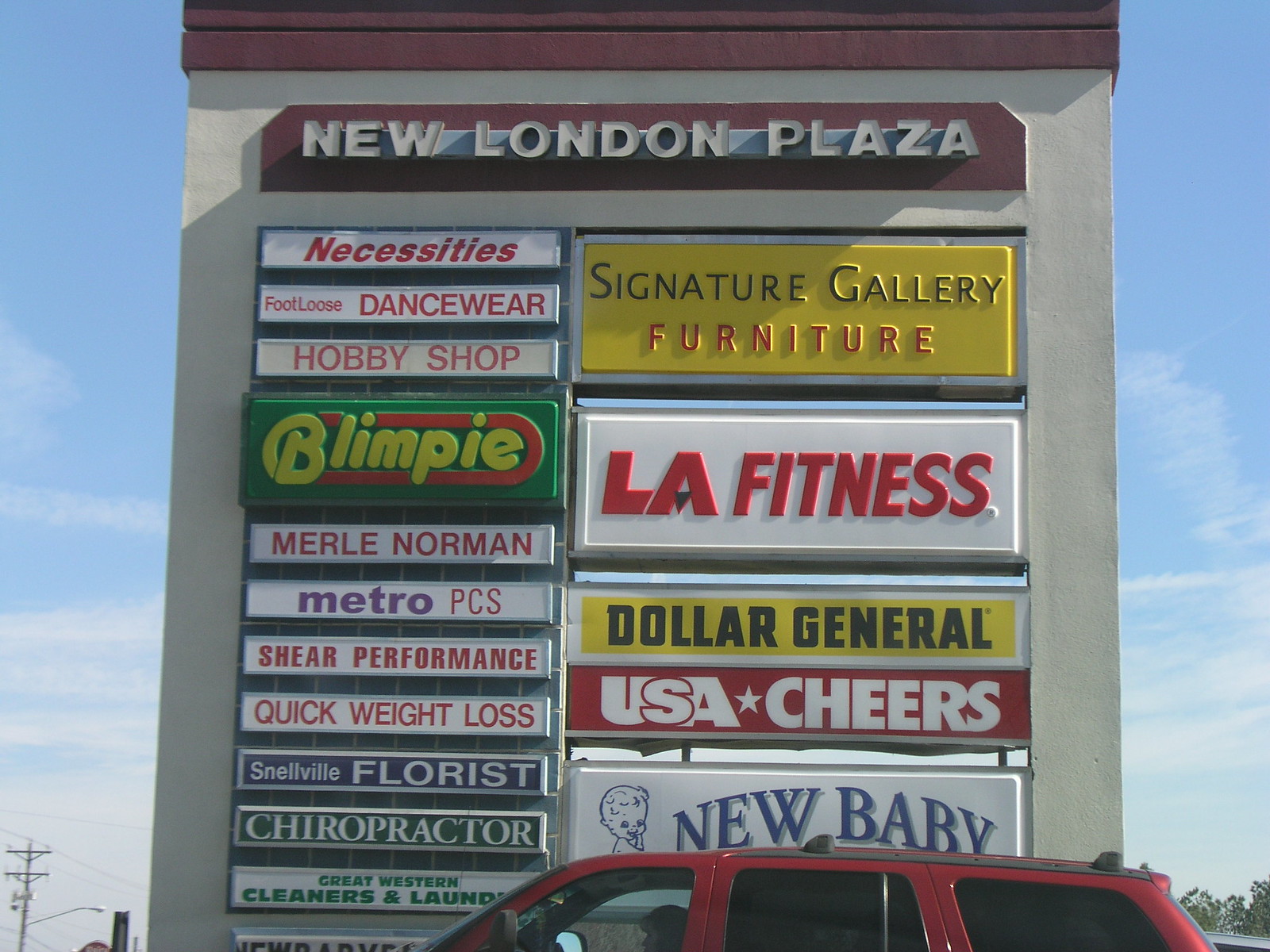The image depicts a large, multicolored sidewalk sign for New London Plaza set against a clear blue sky. The main background color is tan with a brown or burgundy stucco top where the plaza name is displayed in illuminated white letters. The sign is approximately 20-25 feet high and 10-15 feet wide, characteristic of those seen in strip malls or shopping centers. 

To the left of the sign is a column listing various store names in smaller, rectangular signs: Necessities, Footloose Dancewear, Hobby Shop, Blimpie (in yellow print against a blue background), Merle Norman, Metro PCS, Shear Performance, Quick Weight Loss, Snellville Florist, Chiropractor, and Great Western Cleaners and Laundry. The right column features larger signs for Signature Gallery Furniture, LA Fitness, Dollar General, USA Cheers, and New Baby Products, indicating either bigger businesses or those that opted for more prominent signage. The sign displays a diverse color range including black, red, green, yellow, blue, and brown.

At the very bottom of the image, you can see a red Jeep with black tinted windows driving to the left. The front driver's side window is open, revealing the silhouette of the driver's head.